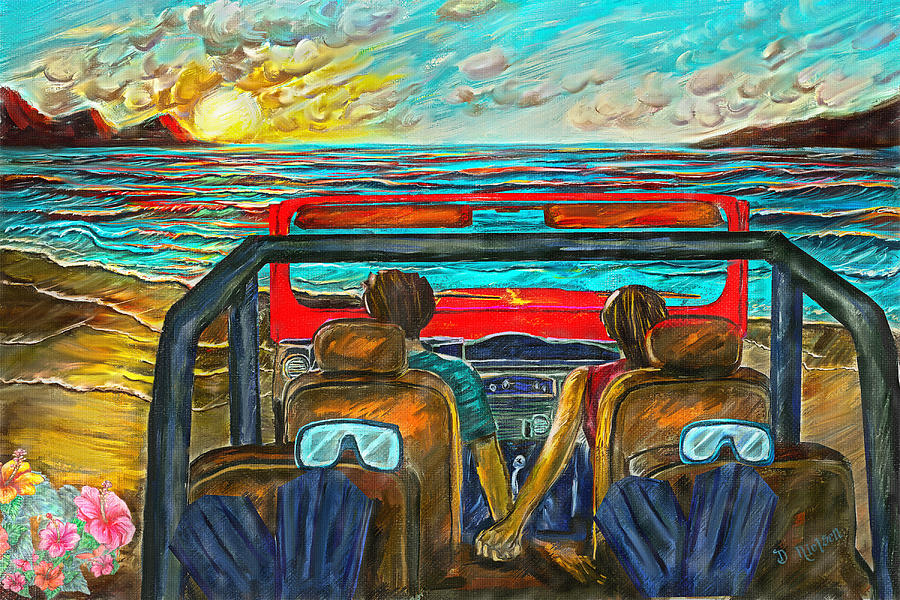The painting captures a vibrant and colorful beach scene, likely created using pastels or oil on canvas. The sky is a blend of blue with white and grey clouds, making way for a distant, yellow sun partially obscured by mountains. Below the scenic sky, a blue ocean with hints of red and orange shading meets a sandy shore.

In the foreground, a jeep with no top and visible red and black colors, as well as brown seats and a roll bar, is parked on the beach. Seated inside are a man in a blue shirt and a woman in a red shirt, both with brown hair, holding hands and gazing at the sunset. Behind them in the jeep, snorkeling gear including two pairs of goggles and grey flippers are carefully placed.

To the bottom left of the composition, there are colorful flowers — pink, green, yellow, and orange — adding a lively touch to the sandy foreground. The artist, D. Nielsen, has signed the painting at the bottom right in grey. The overall scene evokes a nostalgic and serene beach experience, perhaps reminiscent of a specific location like the island of Kauai.